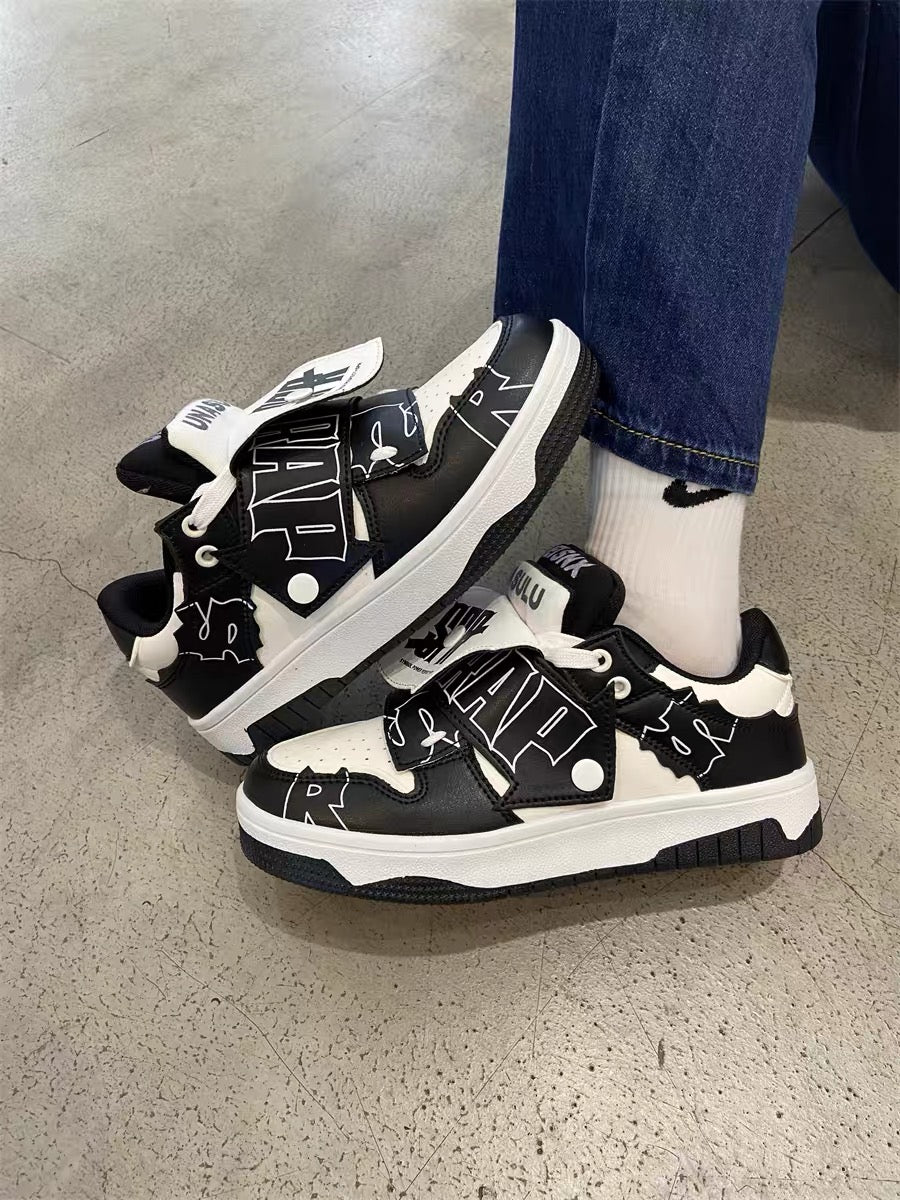This photograph captures a detailed view of a person's left foot, dressed in blue jeans that are slightly hiked up and a white sock featuring a black Nike swoosh. The scene is set on an off-white and black linoleum floor with visible lines and texture. The focal point is a pair of black and white leather sneakers, distinctive for their puffy appearance and flat, moon suit-like sole. The left shoe is worn on the person's left foot, while the right shoe leans against their left shin. Both shoes feature a uniquely designed tongue, which is snapped in and partly conceals the laces. Markings on the shoes include the letters "ULU" and "R," possibly indicating a special or collector's item, though the brand remains uncertain.